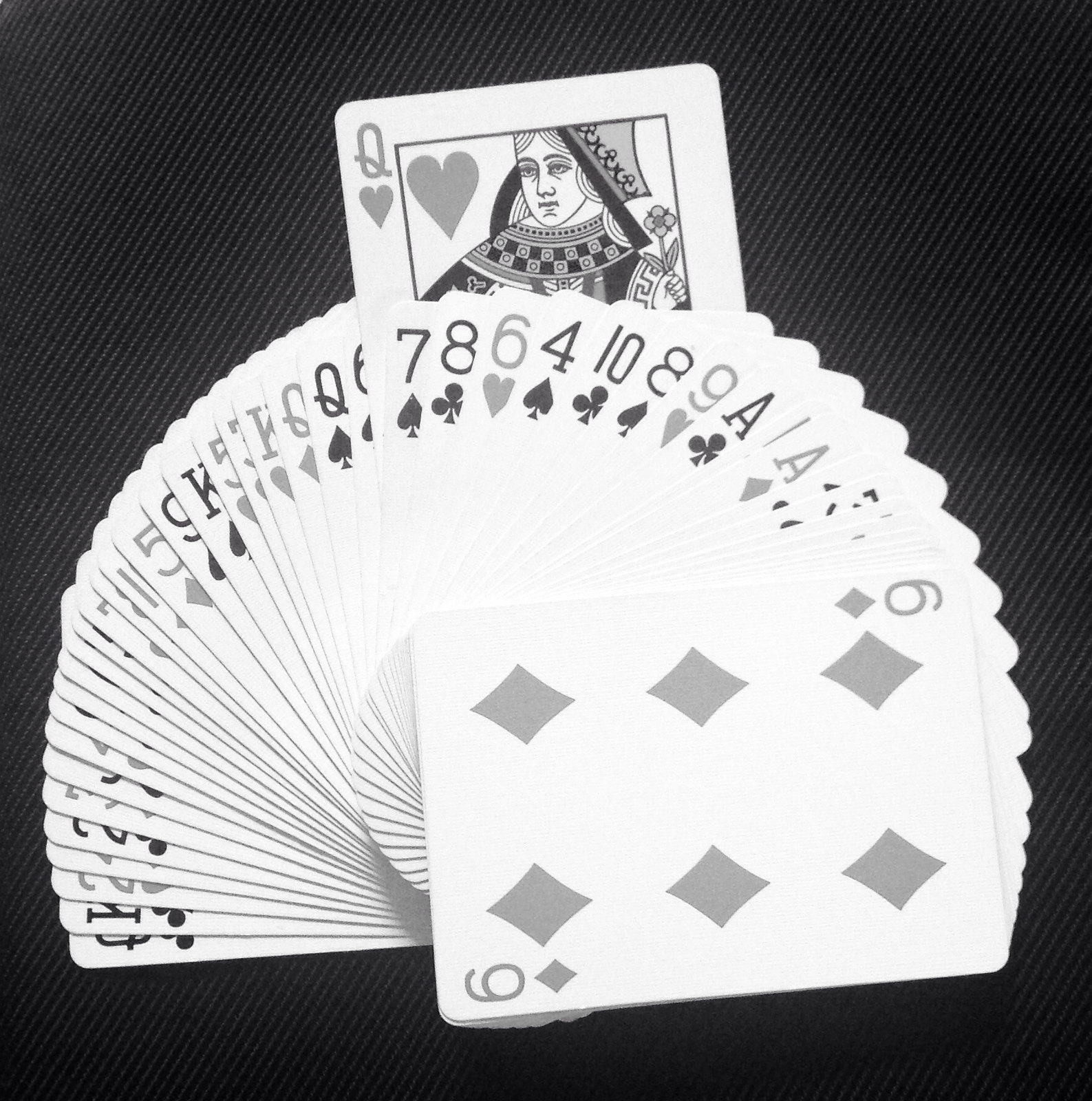The image captures a deck of cards splayed out in the fashion of being held in one’s hand, where the bottoms of the cards are close together while the tops fan out to display the numbers and suits in the corners. The cards are not in any specific order and appear to be randomly arranged. The photograph is rendered in black and white, limiting the visual palette to shades of gray.

Amidst the spread, the Queen of Hearts is prominently pulled out from the center, showcasing her classic depiction complete with a regal headdress and a large checkerboard collar. The background of the image is dark, possibly indicating that the cards are resting on a mat or table surface.

On the far right end of the deck, the Six of Diamonds is facing up, while the opposite end reveals the Queen of Clubs followed by the King of Clubs, a Two, a Four, and another Two. Most of the cards are partially obscured by others, making some of their details indistinguishable. Directly beneath the partially pulled Queen of Hearts, cards in view include the Seven of Spades, Eight of Clubs, Six of Hearts, and Four of Spades.